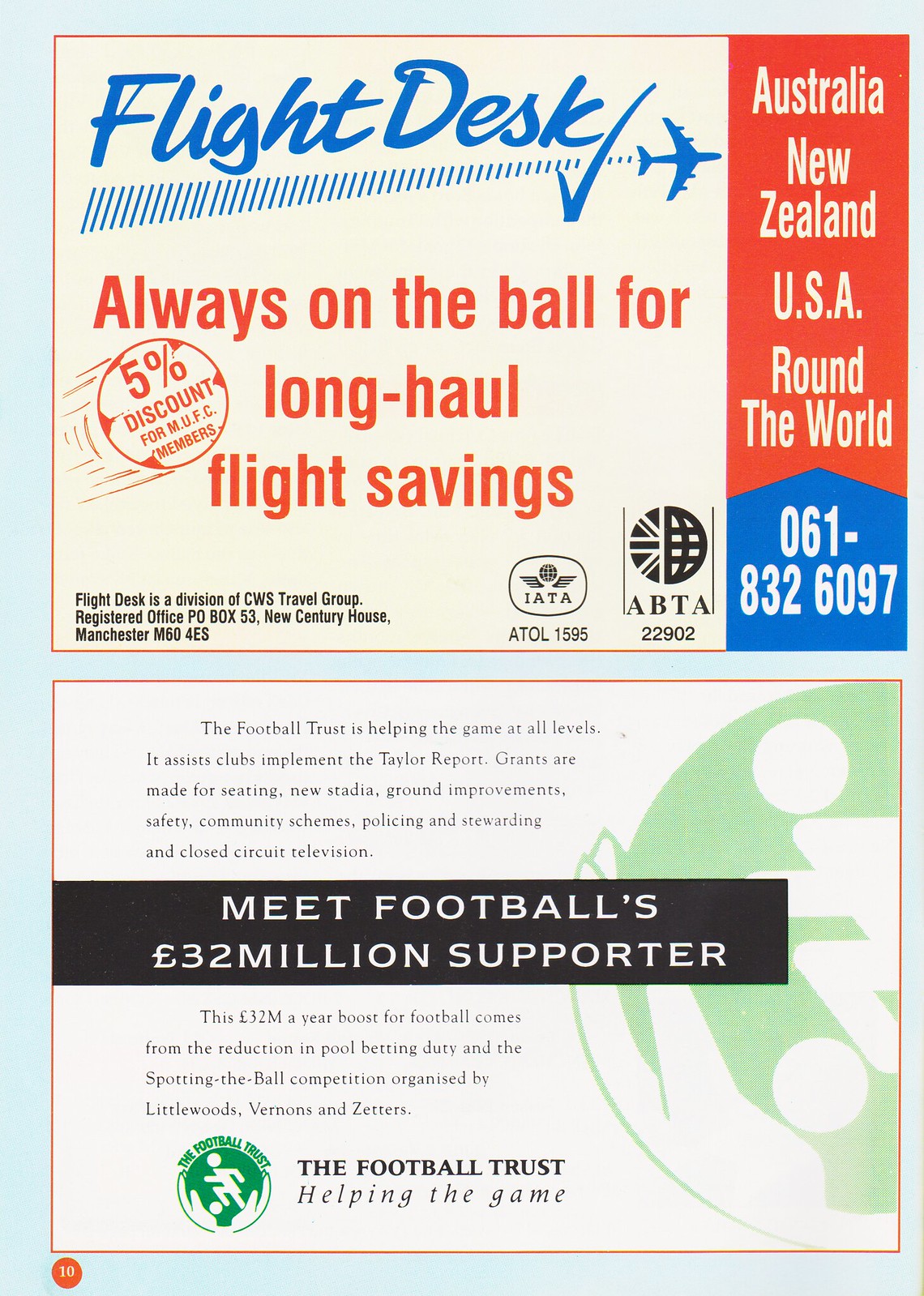In this image, there are two distinct advertisements placed one above the other. The top half is an advertisement for Flight Desk, predominantly featuring a cream background. A prominent blue font spells out "Flight Desk" with an image of an airplane trailing vertical lines, resembling a gasoline trail, moving towards the right. Below this, red text reads, “Always on the ball for long haul flight savings,” accompanied by a checkmark behind the airplane. A circular icon on the left states a “5% discount.” The right side of the advertisement has a red and blue border displaying the white text: “Australia, New Zealand, USA, around the world,” and a blue phone number, 061-832-6097. Below, smaller black text and logos, including IATA and ABTA, provide additional information.

The bottom half showcases a promotional black banner with white text stating, "Meet Football’s 32 million pound supporter," part of a Football Trust campaign. Further black text on a white background explains that this significant financial support results from a reduction in pool betting duty and contributions from Littlewoods, Vernons, and Zetters' Spotting the Ball competition. An icon of a soccer player appears to the left on a green background, with additional details surrounding the Football Trust’s mission: to aid football at all levels by assisting clubs, implementing the Taylor Report, improving stadia, security measures, and community schemes. The advertisement concludes with the Football Trust's logo, proclaiming, “The Football Trust helping the game.”